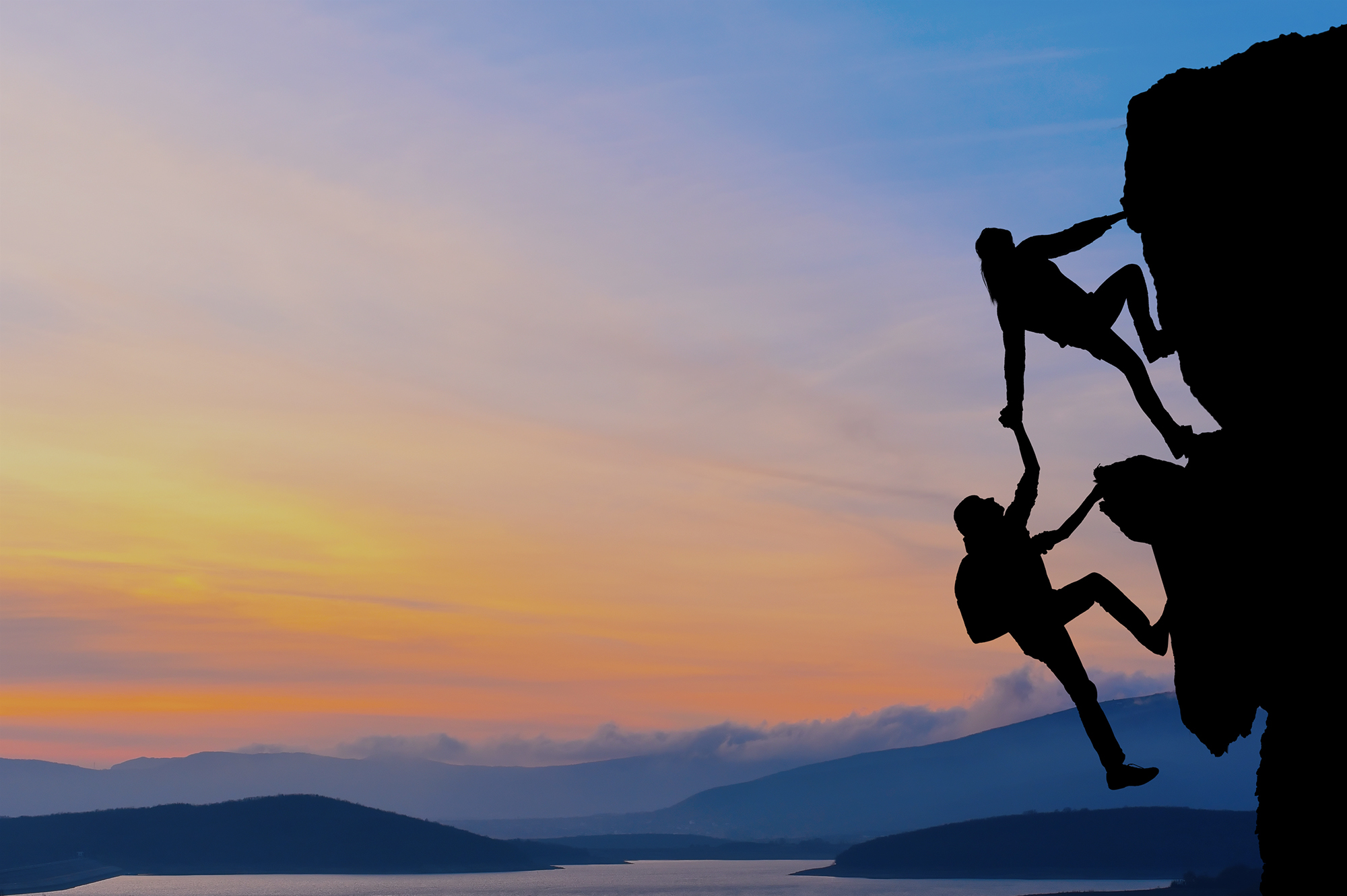In this color photograph taken at sunset, two silhouetted figures are captured climbing a rugged mountainside on the right side of the image. The climbers appear to be without safety gear, enhancing the dramatic nature of their ascent. The person at the top, possibly a woman with a ponytail, reaches down to grasp the hand of the climber below, helping them scale the rocks. Both figures wear backpacks, indicating their adventurous journey. The sky above transitions smoothly from light blue at the top, through purplish white, to brilliant shades of yellow and orange closer to the horizon. In the background, rolling, darkened hills reminiscent of the Appalachian Mountains stretch out, fading into the distance. The scene also includes a serene lake at the bottom of the frame, adding to the image's tranquil yet captivating atmosphere.